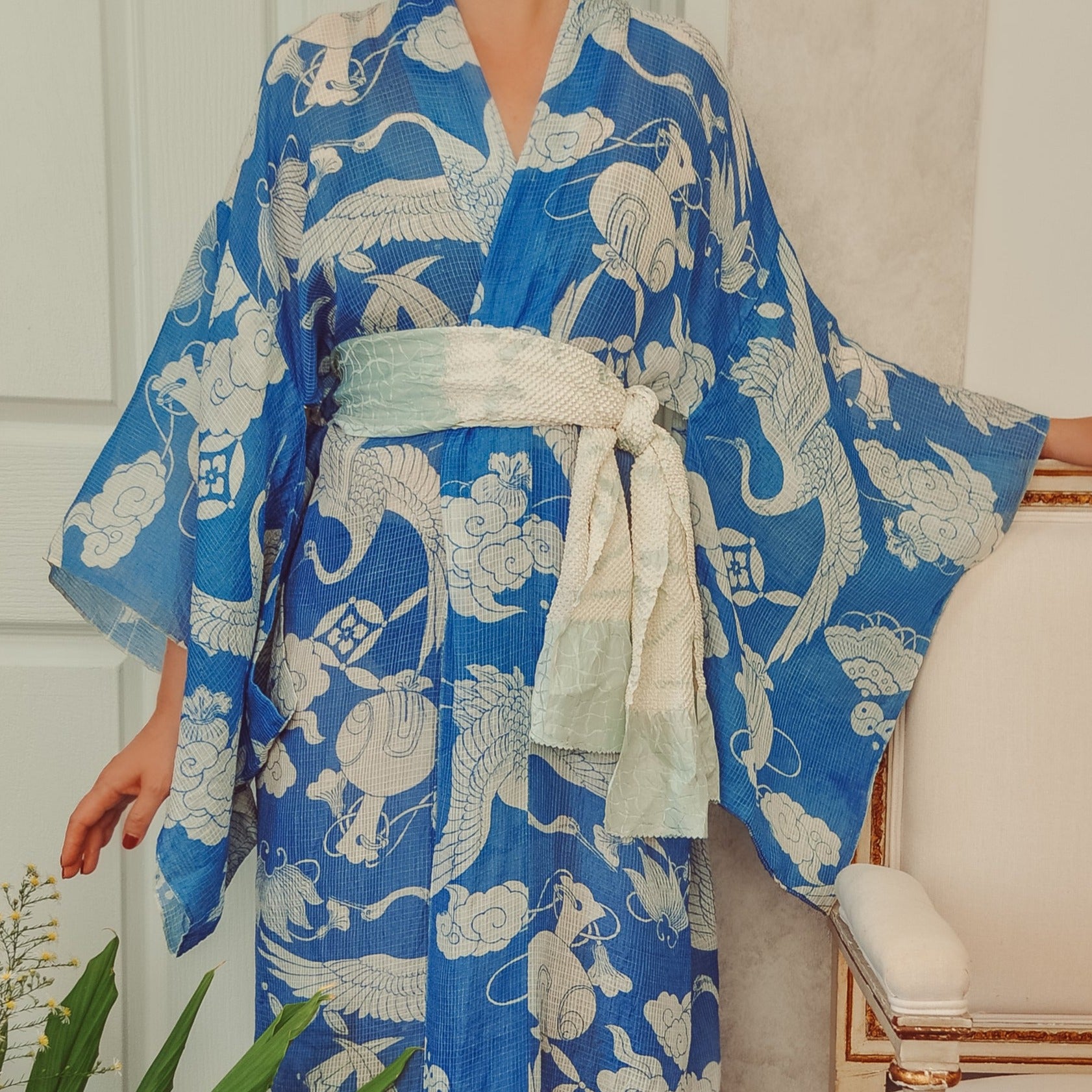In this detailed fashion photograph, a model dressed in a striking kimono poses against a cream-colored background. The kimono is a sky blue adorned with white traditional Japanese imagery, including cranes, stylized clouds, and various ceremonial objects. The garment is cinched at the waist by a wide, light blue and white sash with an indistinct pattern that is intricately tied at the side. The model's right hand, with visible red nail polish on the thumb, rests gracefully by her side, while her left hand is positioned off-screen on what appears to be a luxurious white chair with brown and gold trim. The frame of the photograph cuts off at the model's neck and extends down to her knees, focusing on the detailed attire and partially obscuring her face. A sprig of yellow flowers alongside a few green leaves peeks into the lower left corner of the image, adding a touch of natural elegance.